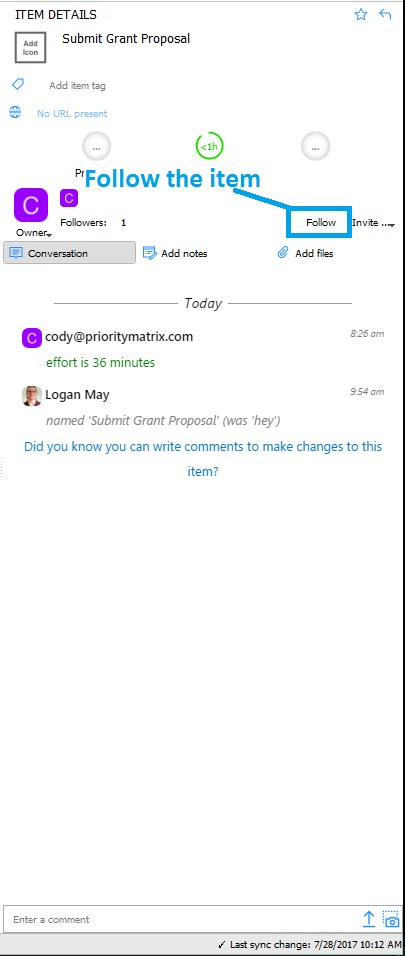**Caption:**

The image showcases a structured layout of a grant proposal submission interface on a white background. At the top-left corner, the title "Item Details" is displayed in black. Below this, the text "Submit Grant Proposal" is prominently featured. An option labeled "Add Item Tag" is accompanied by an icon to its left. Further down, a web-related icon appears beside blue text stating, "No URL Present." Another line of blue text reads "Follow the Item," with a highlighted section around the word "Follow," suggesting an interactive element.

Directly beneath "Follow the Item," there are two purple squares, each containing a white "C," with one square being larger than the other. A third purple square with a "C" is located further down the page. Below these elements, the text lists various items in succession: "Owner," "Followers," "One," "Conversation," "Add Notes," and "Add Files."

The section at the bottom shows an entry logged as "Today" by Cody from PriorityMatrix.com, indicating an effort of 36 minutes. A subsequent comment from Logan May specifies the name of the item as "Submit Grant Proposal" and includes a prompt in blue text advising: "Did you know you can write comments to make changes to this item?"